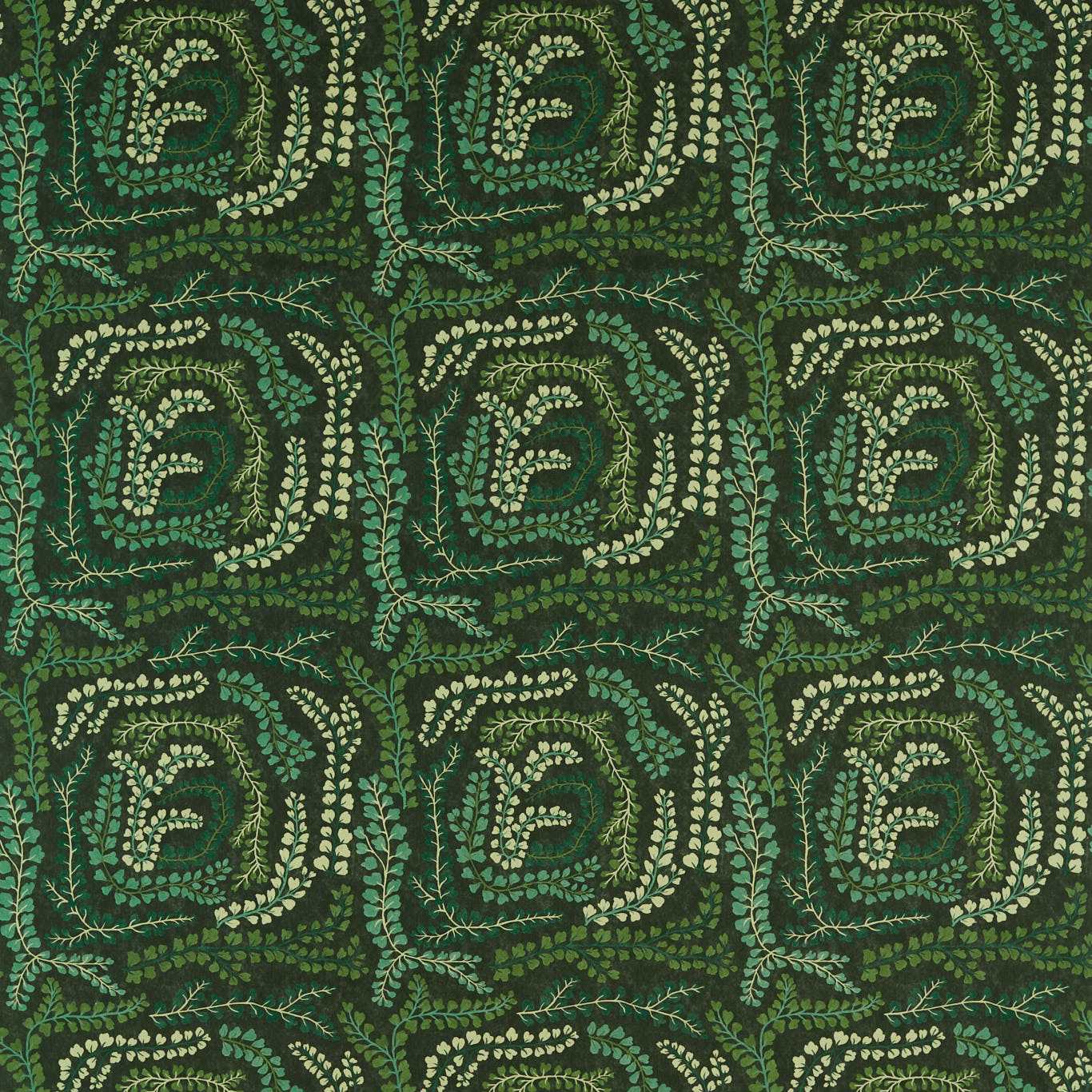The image showcases a detailed, repeating pattern predominantly in shades of green, with intricate botanical designs. The pattern consists of nearly square yet rounded designs arranged in rows and columns—three full rows can be seen, with a partial fourth row at the bottom. Each design features the motif of plant fronds that form a circular pattern, suggesting a floral or leafy appearance. The borders of these square-like designs display various greens and lighter hues, intertwined with branches, leaves, and possibly small flowers. In the center of each design, a form resembling the letter "F" with a protrusion on the upper left side is visible, adding complexity to the overall motif. The entire arrangement gives a textured, almost three-dimensional feel, as if the plants are delicately drawn or woven into the fabric.